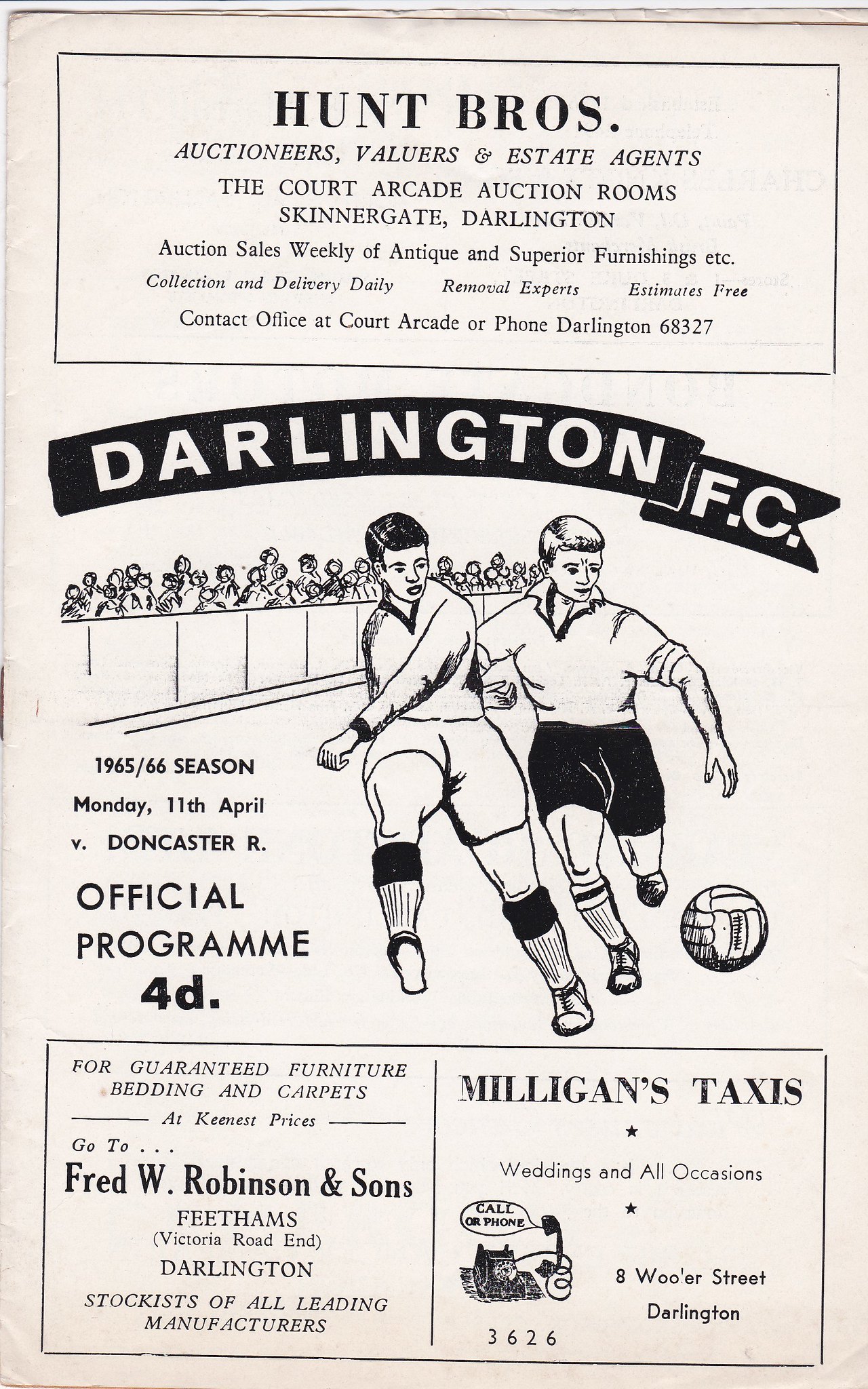This image depicts the official program cover for Darlington FC's 1965-66 season, specifically for their match against Doncaster Rovers on Monday, April 11th. The cover features a prominent ad at the top for Hunt Brothers, Auctioneers, Valuers, and Estate Agents, highlighting their Court Arcade auction rooms in Skinnergate, Darlington. Centrally, a black banner with white text reads "Darlington FC," flanked above by an old-school advertisement for Hunt Brothers' services, including antique and superior furnishings auctions. Below the banner, a primitive yet effective hand-drawn illustration shows two soccer players vying for the ball, with a crowd of spectators and fencing in the background. Text to the left of this illustration details the date, opposing team, and confirms its status as an official program. At the bottom, two additional advertisements are displayed. One promotes Fred W. Robinson and Sons, offering guaranteed furniture, bedding, and carpets at keen prices, and the other advertises Milligan's Taxis, highlighting their services for weddings and all occasions, with an illustration of a corded phone and the contact number 3626. The background of the program has a cream-colored, aged appearance, adding to its vintage charm.